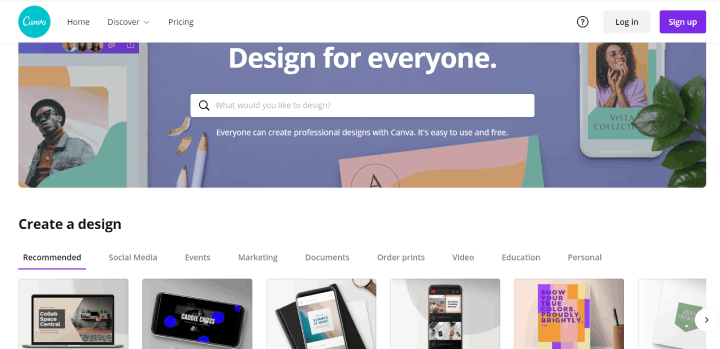This screenshot depicts a web page with a teal blue logo featuring white text at the top left corner. The navigation bar, stretching across the top, includes the options "Home" and "Discover" with a small arrow beneath it, followed by "Pricing." To the far right, there is a circle with a question mark, alongside "Login," and a prominent purple "Sign up" button. Below the navigation bar, a light purple rectangular banner spans the width of the page, adorned with the slogan "Design for everyone."

On the left side of the banner, there is an image of a man displayed as though on a smartphone, accompanied by a couple of lavender pencils. In the center, there is a large white search bar. Various colorful cards in shades of pink, teal, and orange are protruding from the search bar area. To the right, there is an image of a smiling woman wearing a pink shirt, with a portion of a ZZ plant peeking into the scene from the right corner.

Below this banner, there is a section titled "Create a design," offering categories for users to click, such as "Recommended," "Social Media," "Events," "Marketing," "Documents," "Order Prints," "Videos," "Education," and "Personal." Further down, there are six square images arranged in a grid-like manner. The first image shows a laptop, followed by several images of cell phones, and then two additional square pictures with different items.